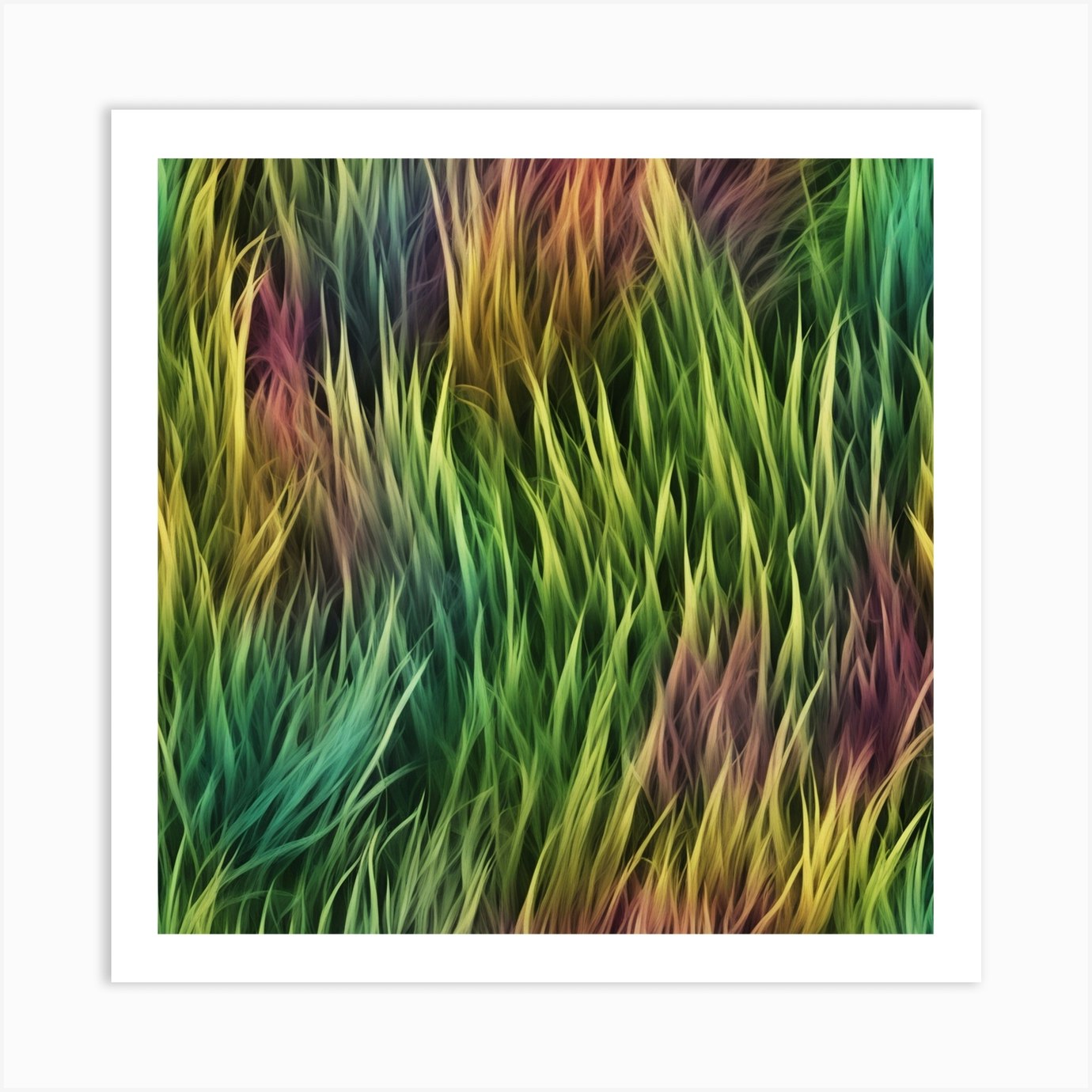This image is a detailed painting framed in white, depicting long, cylindrical blades of grass swaying gently as if caressed by a breeze. The painting radiates vibrant colors, with the predominant green and light green hues interspersed with clumps of pink, light red, blues, yellows, golds, and oranges. The gradient shading gives the blades a dynamic, prism-like effect, where the tips are lighter than the base. The entire frame is filled with these feathery, multi-colored grasses, creating a beautiful and mesmerizing scene that captures the natural motion and diverse palette of the grass. The close-up perspective and hand-painted details add to its intricate, almost quilt-like appearance, making it a truly captivating piece of art.